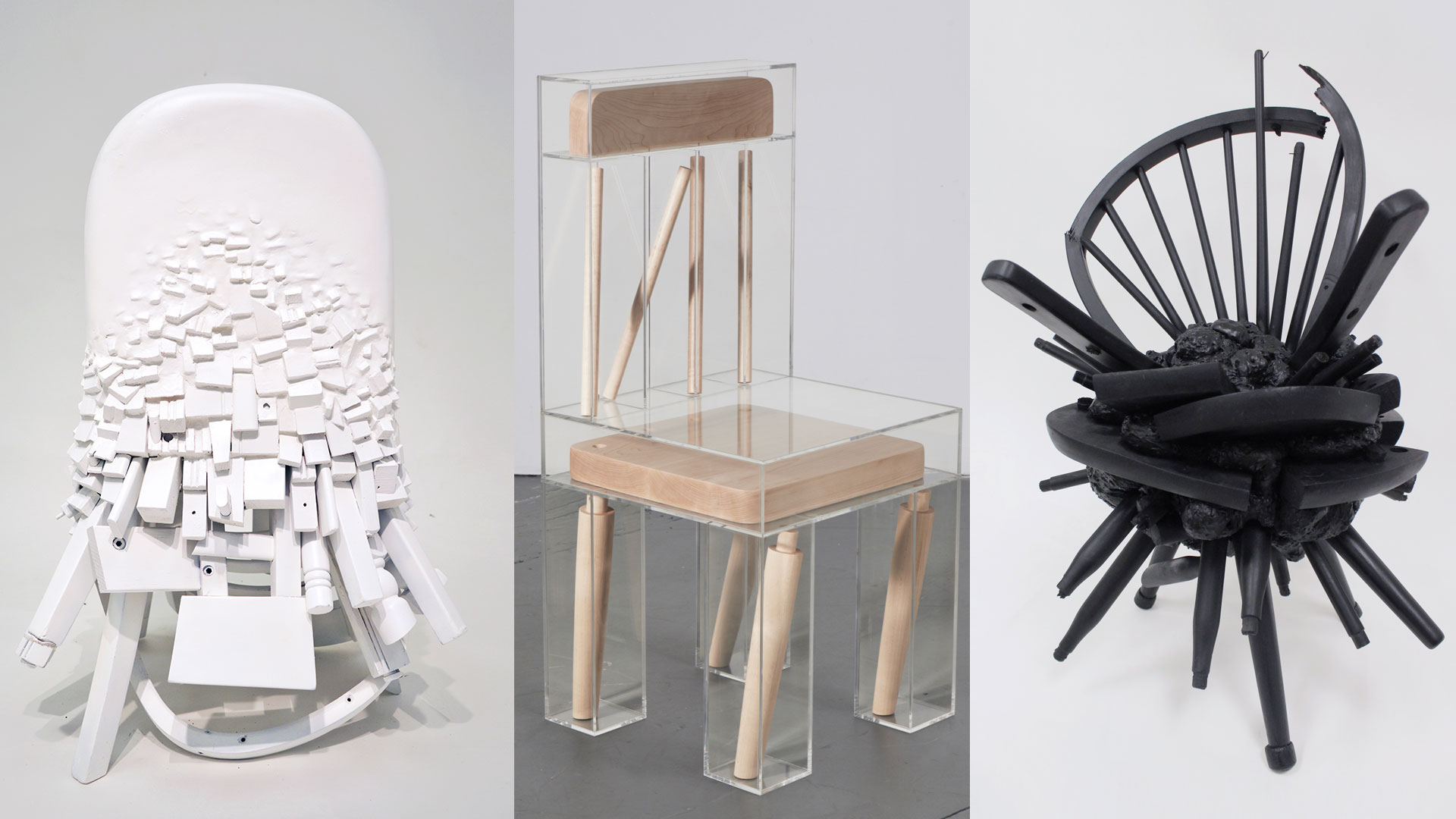The image showcases three professionally photographed, modern art sculptures of chairs, each with unique and abstract designs against a neutral, off-white background. 

The first chair sculpture resembles an oval white pill that erupts into a chaotic assembly of squares jutting out from its form. This piece exudes an abstract aesthetic with its dynamic, fragmented structure.

The middle sculpture is a conventional wooden chair that appears disjointed and fragmented, with its components encapsulated within clear plastic or plexiglass rectangles. The wooden elements, including spindles and legs, seem to hover within these transparent casings, creating an illusion that they are not held together by screws but by the fused plexiglass. The seat is notably a cutting board, contrasting with the polished wood and clear plastic features.

The final sculpture features an intricate and abstract assemblage of black cylinders, spikes, and shapes. This cluster is composed of numerous neutral-shaded elements, forming a complex and visually engaging piece. Its abstract nature and the interplay of various geometric forms evoke curiosity and interpretation.

Each sculpture transforms the traditional concept of a chair into a distinct and imaginative work of modern art.